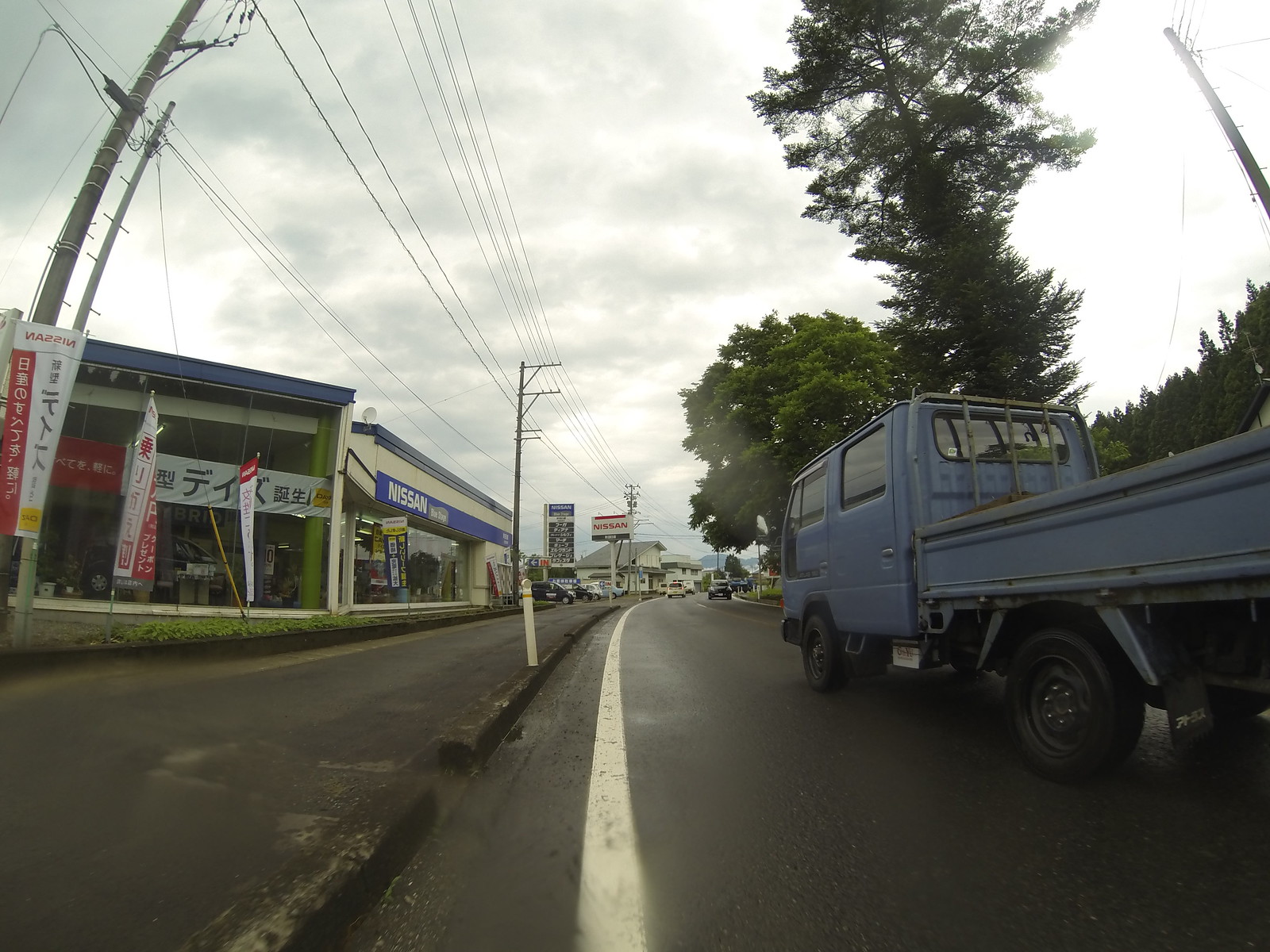In this image, a bustling street in a foreign country is captured in vivid detail. The concrete roadway features white street markings and hosts a variety of traffic, including a distinctive blue, old-style pickup truck with a long cab and black tires. Tall trees with lush, green foliage line the street, adding a touch of nature to the urban setting.

To the left, a prominent Nissan dealership stands out, its name clearly emblazoned on the building’s facade. Additionally, several other buildings and their billboard signs are visible, situated along the sidewalk. Tall wooden poles supporting black power lines stretch across the street, adding a web of connectivity to this lively scene.